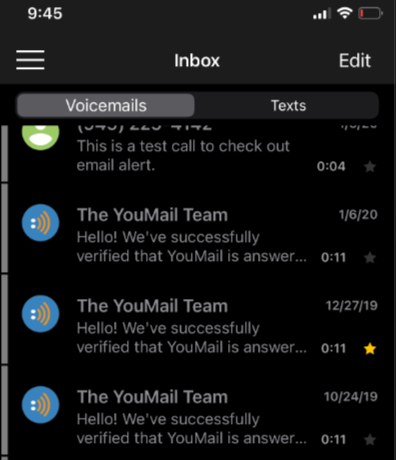The image depicts a black screen displaying the time as 9:45 in white digits. At the top, the screen is labeled "Inbox" and "Voicemails," along with several timestamps. The first entry showcases the icon for an incoming call accompanied by a green symbol. This entry states, "This is a test call to check out email alert," recorded at 00:04 hours. Below this, three entries are preceded by round blue icons indicating incoming calls. These entries reference the email team, stating, "Hello, we've successfully verified that email is answering." The dates for these entries are formatted in day/month/year: 06/01/2020, 27/12/2019. One of these entries features a gold star, the significance of which is unclear. Overall, the screen appears to document successful email verification processes.